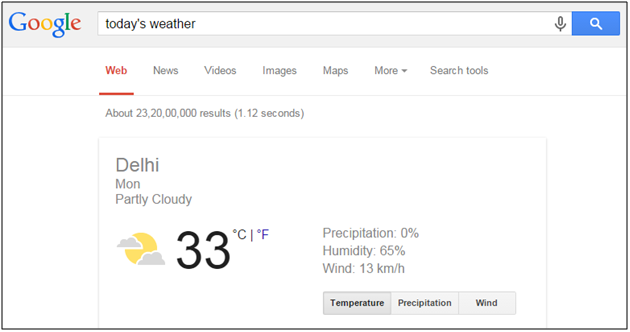The image is a detailed, colorful landscape screenshot showcasing a portion of someone’s desktop or laptop screen. Centered prominently on the screen is the classic Google website, instantly recognizable by its iconic logo displayed in the upper left corner. The logo features the familiar sequence of colors: a blue "G," followed by a red "o," a yellow "o," a blue lowercase "g," a green "l," and a red "e." Below the logo, the search bar is visible, indicating the user has typed in "today's weather." 

The search results reveal current weather conditions for Delhi: it’s Monday, the skies are partly cloudy, and the temperature is 33 degrees Celsius. Further details include zero percent precipitation, 65 percent humidity, and a wind speed of 13 kilometers per hour, suggesting that the query was made by someone in or interested in the weather of Delhi. 

On the right, there are options to toggle between temperature, precipitation, and wind, with the temperature setting currently selected, hence the specific weather details displayed. Additionally, the familiar Google search options are visible across the top: Web, News, Videos, Images, Maps, More, and Search Tools.